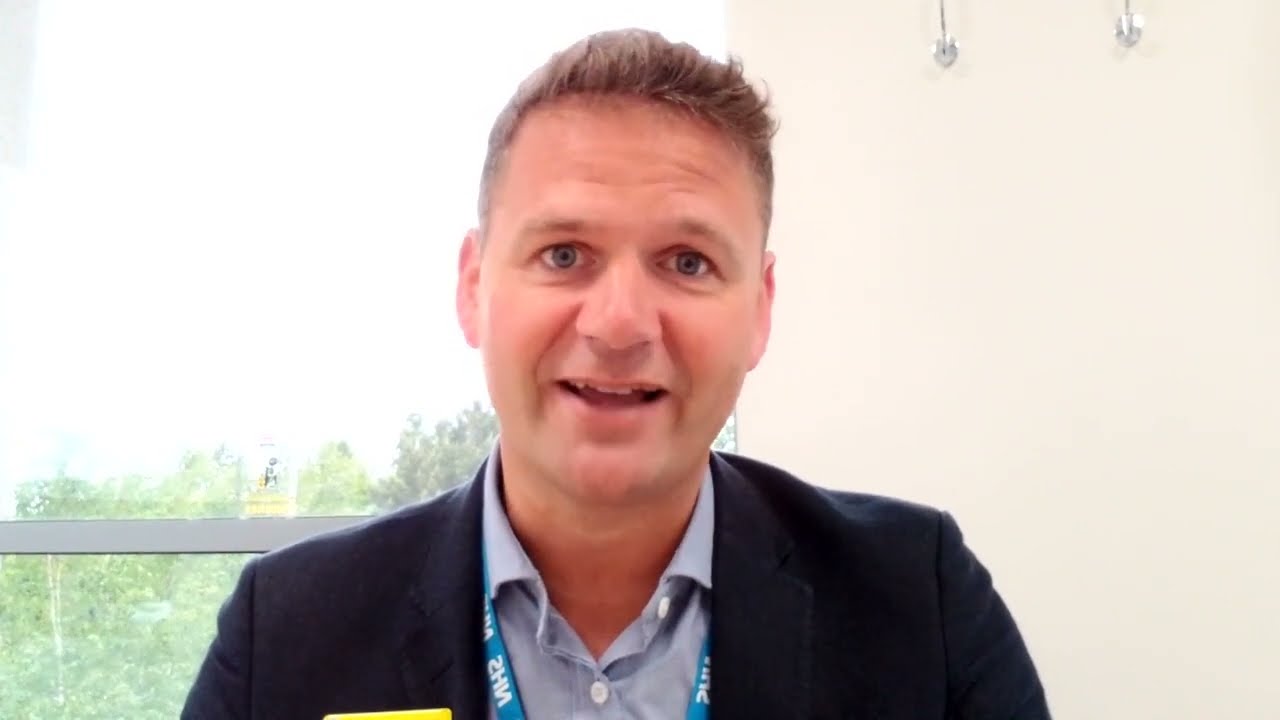The image is a horizontally rectangular photograph capturing a Caucasian man with short, light brown hair, appearing to give a talk. He is looking directly into the camera, with a warm, mid-speech smile showing his top front teeth. He has blue eyes and is dressed in a black suit jacket over a light blue, open-collared button-up shirt, with a blue lanyard around his neck displaying the letters "NHS." The photograph is taken indoors, and the man is seated in the corner of two walls. 

To his right is a white wall with two silver coat hooks in the upper corner. To his left, behind him, is a window with a white sill, revealing a bright, white sky and a tree line at the bottom. The light streaming through the window illuminates his face, contributing to the cheerful atmosphere of the image.